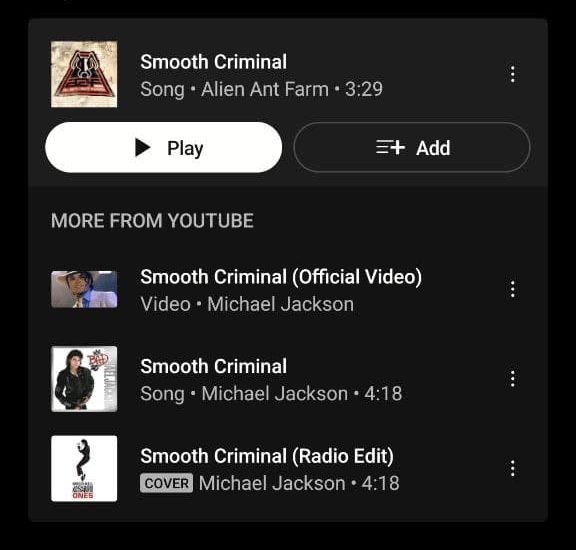The image appears to be a screenshot of a YouTube video interface displayed within a black box. At the very top left, there's an icon featuring an illustration resembling an ant inside a red triangle. Adjacent to this icon, the text "Smooth Criminal" is written in white. Below this, text reads "Alien Ant Farm" followed by a dot and the duration "3:29."

Beneath the title, a white "Play" button is displayed with black text. To the right of the play button, there are three lines with a white plus sign, labeled "Add."

Further down, in gray text, there's a heading indicating "More from YouTube." This section features an image of Michael Jackson with text that reads "Smooth Criminal (Official Video)" and "Video: Michael Jackson." Below, there's another entry with "Smooth Criminal" and in parentheses "Radio Edit - Cover" with the text "Michael Jackson 4:18," displaying a figure striking a pose reminiscent of Michael Jackson's style next to some additional text.